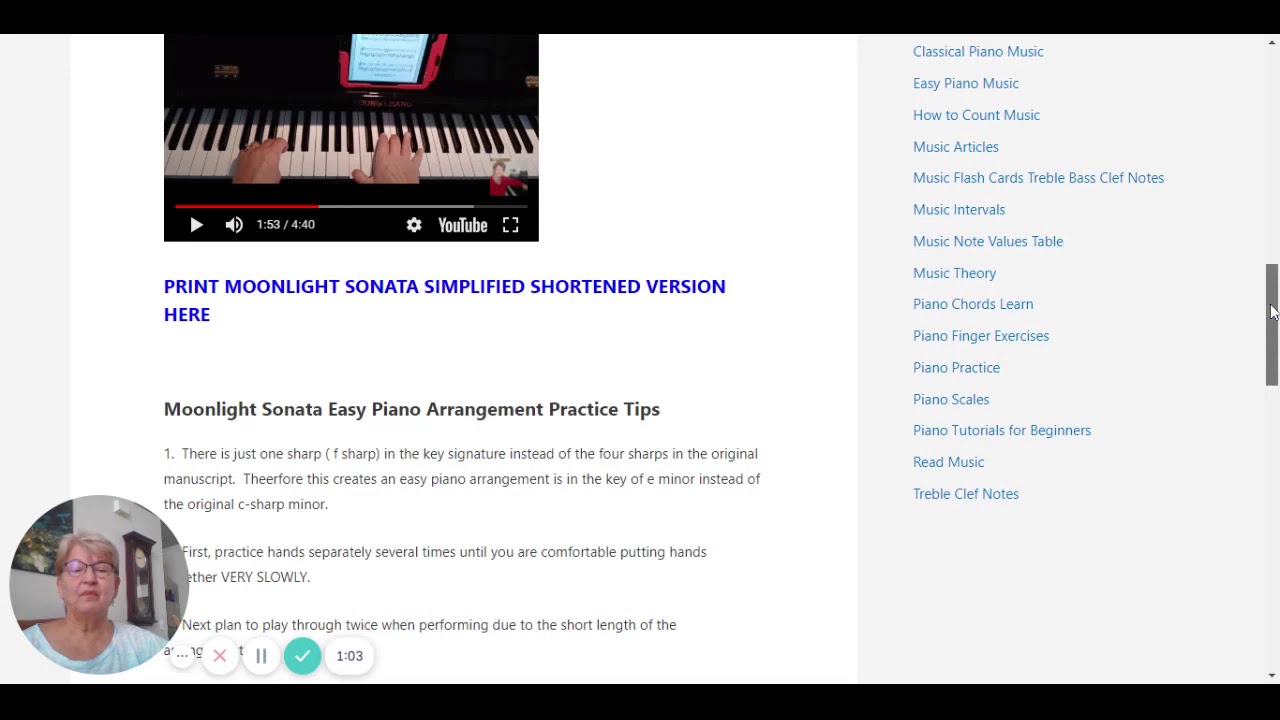In the upper right-hand corner of the webpage, there are several clickable options listed in blue text. From top to bottom, they include: "Classical Piano Music," "Easy Piano Music," "How to Count Music," "Music Articles," "Music Flashcards," "Treble, Bass, Clef Notes," "Music Intervals," "Music Note Values Table," "Music Theory," "Piano Chords Learned," "Piano Finger Exercises," "Piano Practice," "Piano Scales," "Piano Tutorials for Beginners," "Read Music," and "Treble, Clef Notes." 

The page is approximately mid-scroll, evidenced by the position of the right-hand scrollbar. The cursor is currently located on the far right side of the screen. 

A YouTube video on the page is paused at 1 minute and 53 seconds, out of a total length of 4 minutes and 40 seconds. Below the video, there is a link labeled "Print Moonlight Sonata Simplified Shortened Version Here."

On the bottom left-hand side of the screen, there is a circular icon featuring an image of a woman. To the right of this image are three symbols: an X (close), a pause button, and a checkmark, followed by a timer reading "1:03."